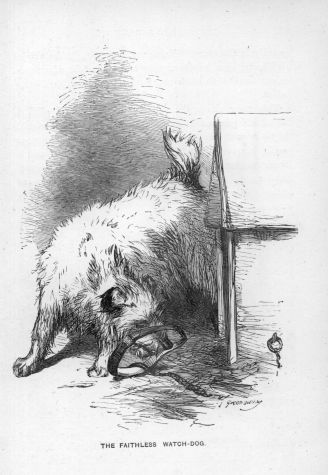This black-and-white sketch, possibly rendered in pencil or charcoal, presents a detailed and somewhat dramatic scene. The main subject is a shaggy dog, depicted with long, stringy hair and a bushy tail, intensely interacting with what resembles a circular object, potentially a bear trap or belt. The dog’s stance and positioning suggest a moment of tension, possibly growling or preparing to attack. Positioned to the right, a portion of a doghouse is visible, complementing the outdoor setting suggested by the composition. The drawing is set against a very light gray paper background, with darker gray shading near the top left, enhancing the depth and contrast. At the bottom of the image, the text "The Faithless Watchdog" is prominently displayed, with an unreadable signature in the lower right corner, adding to the artwork’s mystique.